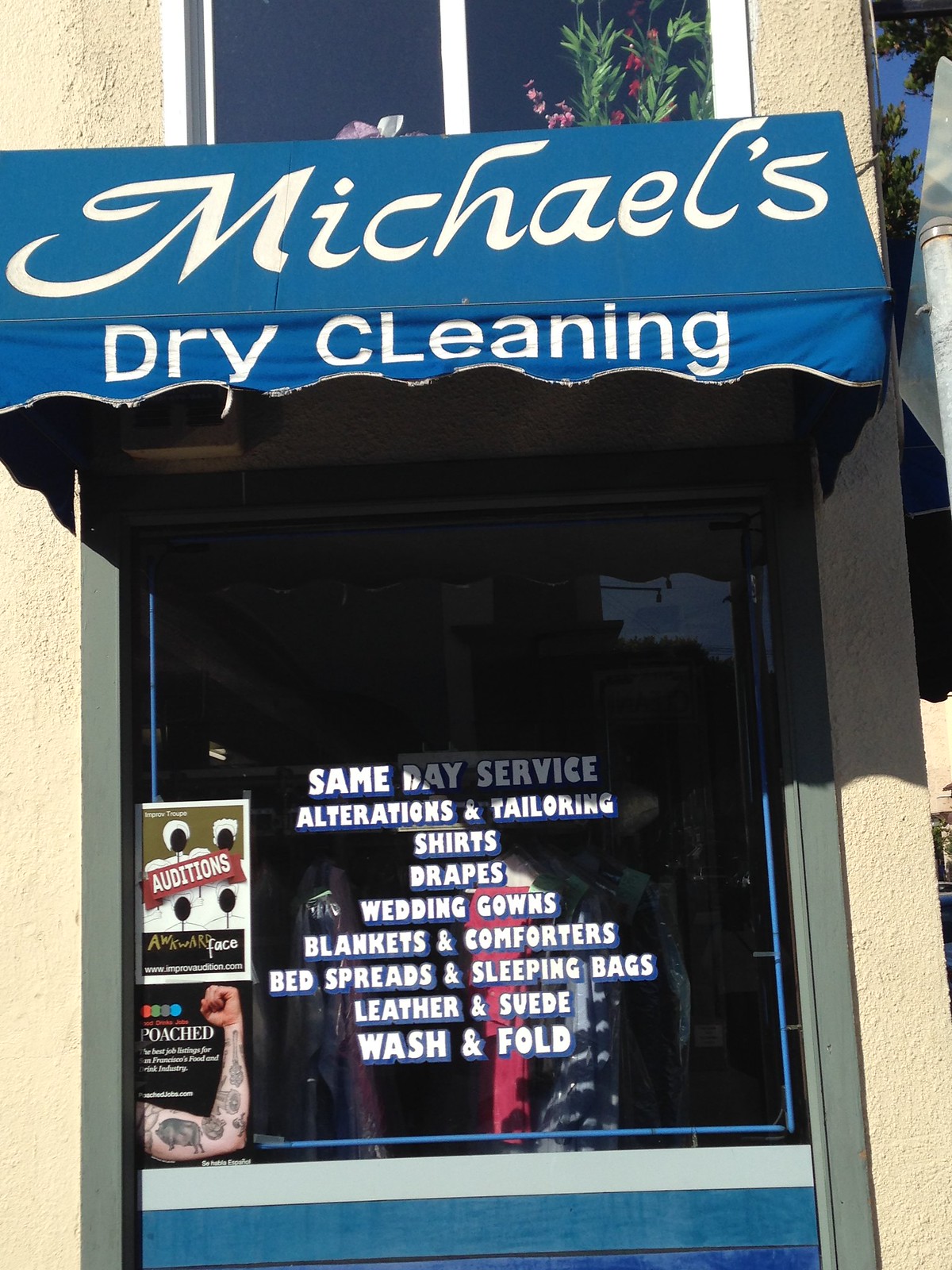This photograph captures the side view of Michael's Dry Cleaning storefront, situated on a corner. Dominating the scene is a large blue canopy above the storefront, emblazoned with "Michael's Dry Cleaning Service" in crisp white font. The storefront's tan stone walls frame a central door, beneath a window that lists the various services offered by Michael's. The bold and capitalized text on the window prominently advertises: "Same Day Service, Alterations and Tailoring, Shirts, Drapes, Wedding Gowns, Blankets, Comforters, Bedspreads, Sleeping Bags, Leather, Suede, and Wash and Fold." Additional signs, likely advertising local events, are visible to the left of the window. The photograph was taken in daylight, giving it a bright and clear appearance. The colors in the image include shades of tan, white, gray, blue, black, green, red, and pink.